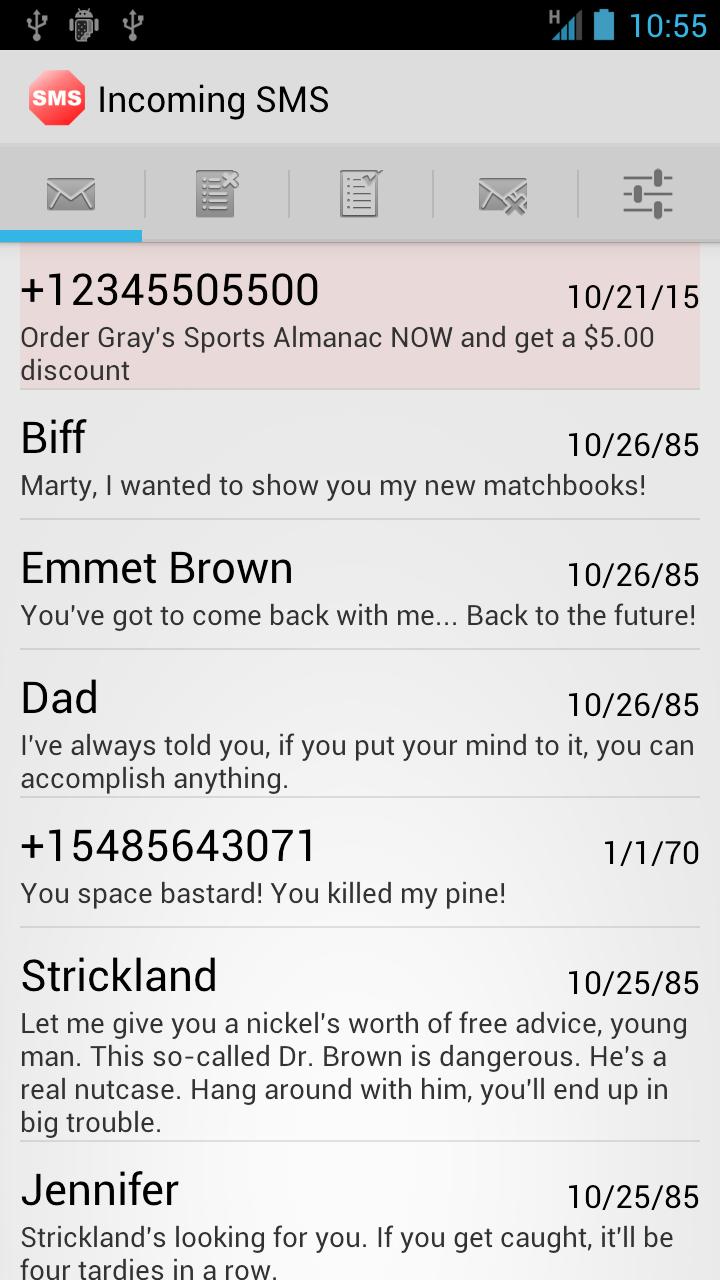The screenshot depicts an Android phone taken at 10:55 with a fully charged battery and a three-bar cellular connection. The screen features a header labeled "Incoming SMS" accompanied by an SMS icon resembling a stop sign with the letters "SMS" in white. Below the header is a taskbar area that houses five different icons, with the first icon resembling a plain letter, likely indicating the mailbox selection.

The interface shows a list of seven SMS messages, each from distinct senders and timestamps:
1. From +12345505500 on 10-21-15: "Order Gray's Sports Almanac now and get a $5 discount."
2. From Biff on 10-26-85: "Marty, I wanted to show you my new matchbooks."
3. From Emmett Brown on 10-26-85: "You have got to come back with me back to the future."
4. From Dad on 10-26-85: "I have always told you if you put your mind to it, you can accomplish anything."
5. From +15485643071 on 1-1-70: "You space bastard, you killed my pine."
6. From Strickland on 10-25-85: "Let me give you a nickel's worth of free advice, young man, this so-called Dr. Brown is dangerous. He is a real nutcase. Hang around with him; you will end up in big trouble."
7. From Jennifer on 10-25-85: "Strickland is looking for you. If you get caught, it will be four tardies in a row."

The user interface appears significantly outdated with a predominantly gray color scheme.